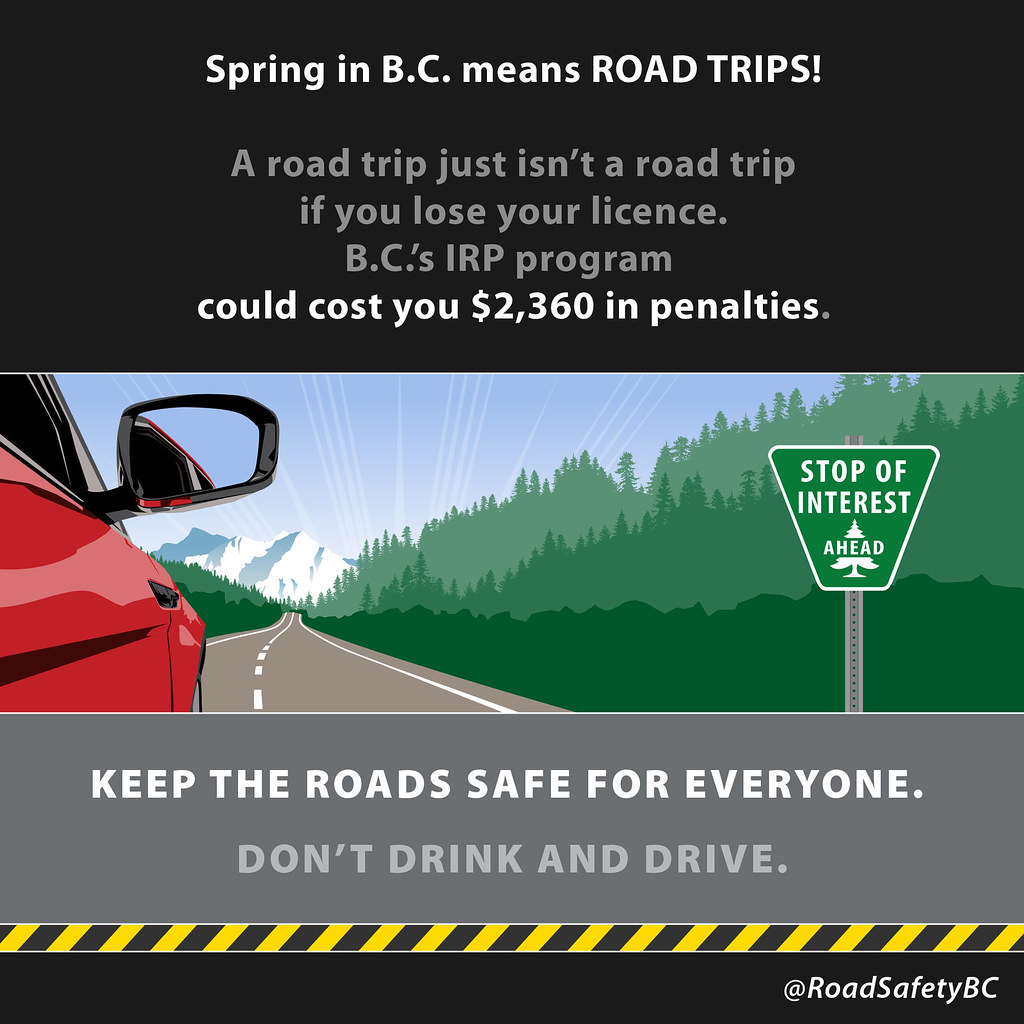The image is a detailed public service announcement in a square format featuring vibrant graphic design and illustration. The top third of the image is a black background with prominent white and gray text, stating: "Spring in BC means road trips! A road trip just isn't a road trip if you lose your license. BC's IRP program could cost you $2,360 in penalties." Below this text, the central portion of the image showcases an illustrated scene: a red car drives along a paved highway through a forested area, heading towards a snow-capped mountain in the distance. On the right side of the road is a green triangular sign reading "Stop of Interest Ahead," with the word "AHEAD" superimposed on a white tree. The bottom third of the image features a gray horizontal strip with white text urging, "Keep the road safe for everyone. Don't drink and drive." Beneath this is a narrow yellow and black diagonal band resembling caution tape. The bottom right corner has the text "Road Safety BC" in white on a black background, marked with an at symbol (@). The image effectively blends illustration with typographic design to convey its important anti-drinking and driving message.